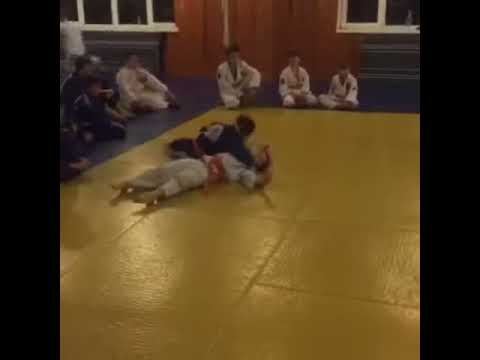In this somewhat blurry image, we observe a karate class for young kids, situated indoors, likely in a dojo during the late evening or nighttime. At the center of the image, two children are engaged in a sparring match on a gold-colored mat. One child, dressed in a blue uniform, appears to have the upper hand, pinning the other child, who is clad in a white uniform, to the mat with an elbow at their neck. This action suggests the child in blue has successfully taken down their opponent. Surrounding the center mat is a blue border mat, atop which several other children, also in karate uniforms of white or blue, are seated and observing the match intently. The backdrop includes walls and windows, accompanied by thick black framing that forms rectangular patterns, contributing to the overall composition of this lively indoor setting. Text is notably absent from the image, but various colors such as yellow, white, red, blue, and black are present, adding vibrancy to the scene.